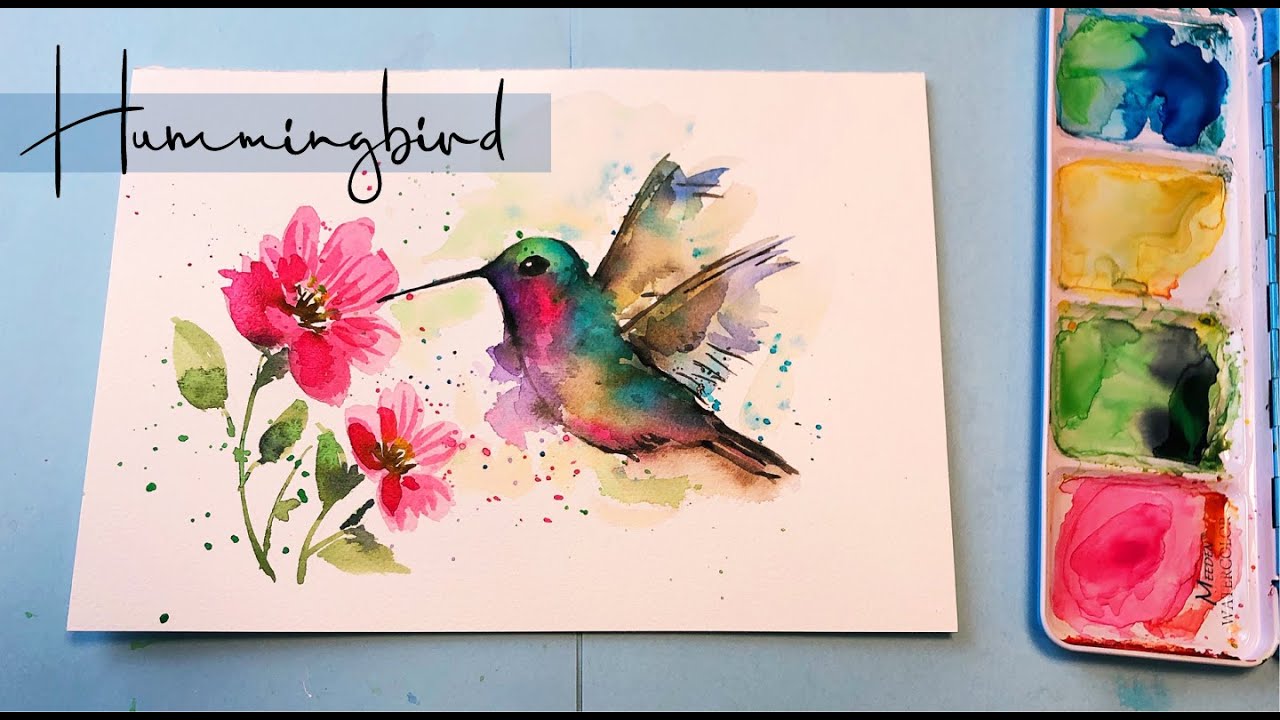The image showcases a detailed painting of a vibrant hummingbird, captured mid-flight as it feeds from two pink flowers. The bird's back is a rich green, transitioning to a reddish area under its chin, with its breast displaying a blend of yellow and pink hues. Its very long, black beak is extended into one of the pink flowers, which stem from a green base. The wings exhibit a mix of colors, predominantly purple. Adjacent to the bird, on the right-hand side of the image, is a painter's palette set against a light blue background, containing the very colors used in the artwork: a pinkish-red, various greens, yellow, mustard, and bluish-green. The composition rests on what appears to be a white card, prominently labeled "hummingbird" in bold black letters. To the right of the label are splotches of the colors featured in the painting, further emphasizing the texture and effort put into this artistic creation.